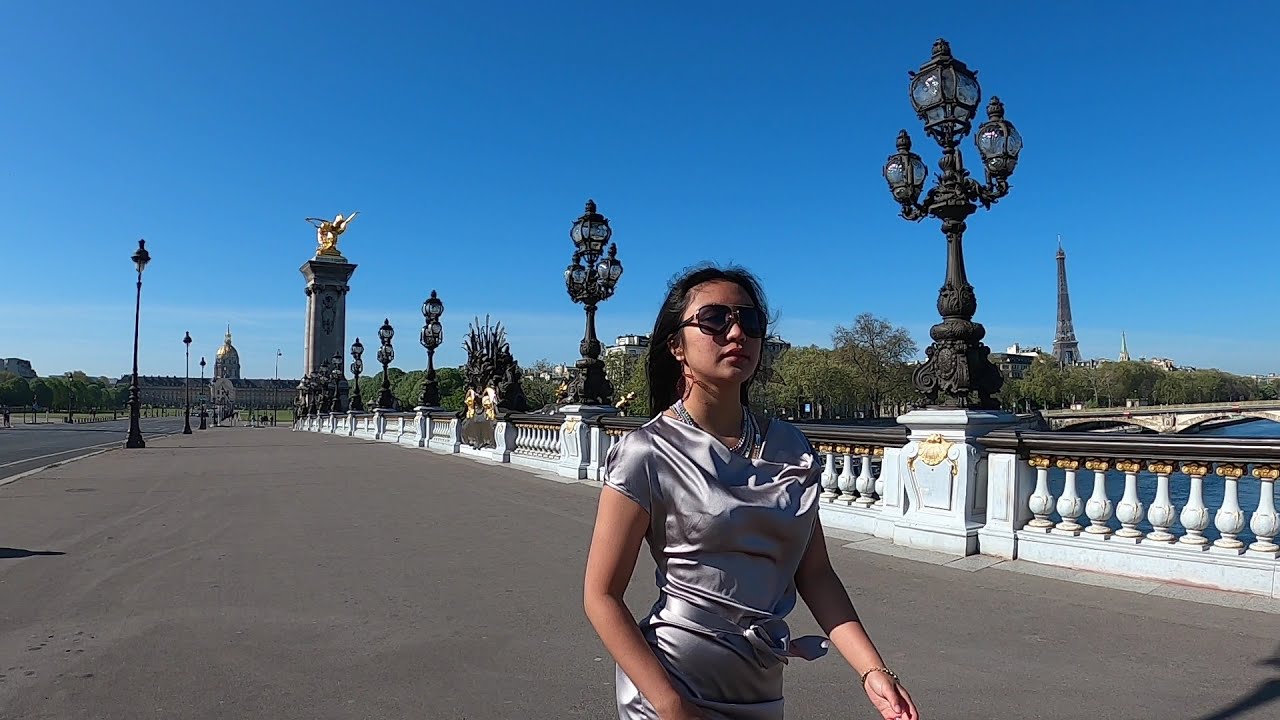The image captures a woman walking towards the camera on a wide, well-paved sidewalk that likely serves as a bridge in a picturesque urban setting. She is dressed in a shimmering silver satin outfit that appears to be coordinated separates of a silky top and bottom or a glittery, tight-fitting dress with a tie around her waist. Her attire is completed with many-stranded necklace and large, dream catcher-like earrings. She sports sunglasses and has long, dark hair flowing behind her.

To her right is a long, ornate white railing with rounded columns, and to her left is the distant road bordered by streetlights. These streetlights are elaborate, candelabra-shaped, with three-tiered bulbs atop pedestals, adding to the bridge's opulence.

Behind her, the Eiffel Tower rises prominently amidst a backdrop of trees and large, significant-looking buildings, one of which is a long rectangular structure adorned with a dome. The scene is bathed in the light of a clear, sunny day with a vivid blue sky overhead, casting half of her face in sunlight and the other half in shade.